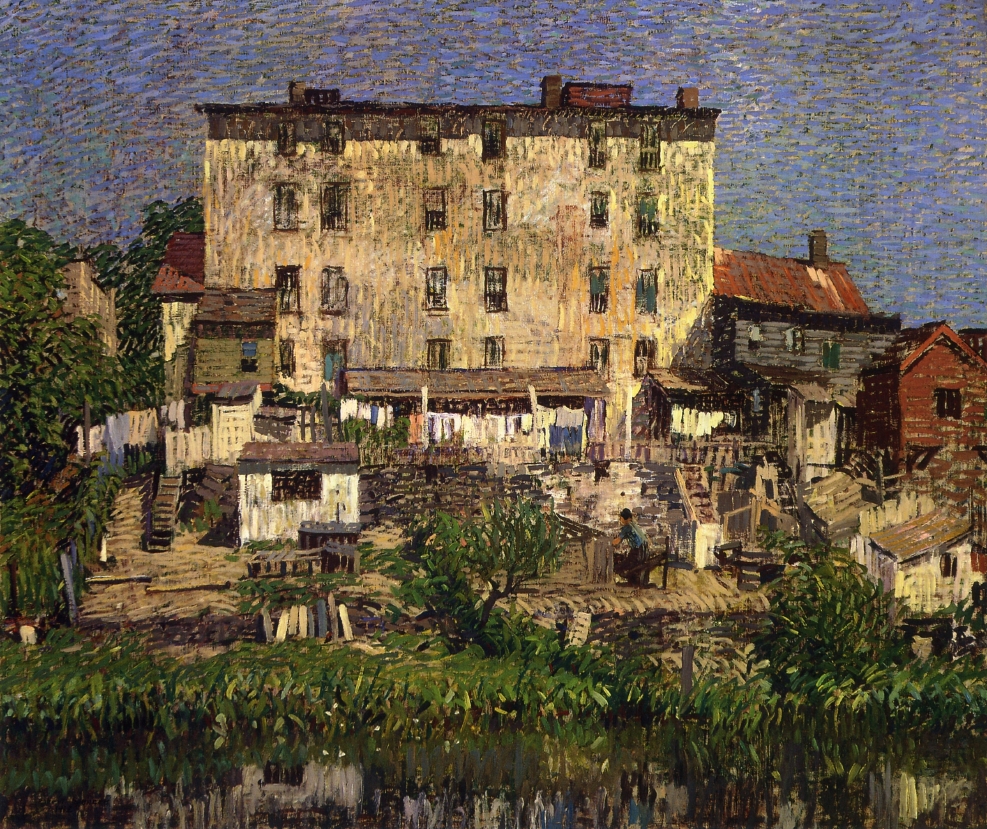This painting depicts a tall, beige, four-story building with numerous brown windows and several chimneys protruding from its dark brown rooftop. In front of the building lies a reflective body of water, possibly a river or lake, bordered by vibrant green grasses and individualized leaves on surrounding trees. To the right of this main structure, there are additional buildings, including a reddish-brown house next to a blue one with a reddish-brown roof, adding to the scene's charm. Interspersed throughout the green shoreline, several small buildings and sheds can be seen, some appearing slightly dilapidated. Clothes hang on a clothesline on the left side of the painting, near a ladder and what seems to be a small shed. There is a person, possibly a man or woman, at the foot of the building, working on something by the ground near the water. The painting style is reminiscent of Van Gogh or Monet, with a sky that blends hues of blue, purple, and gray. Overall, this artwork beautifully captures the serene and somewhat neglected essence of a historic, multi-story building amidst its picturesque surroundings.